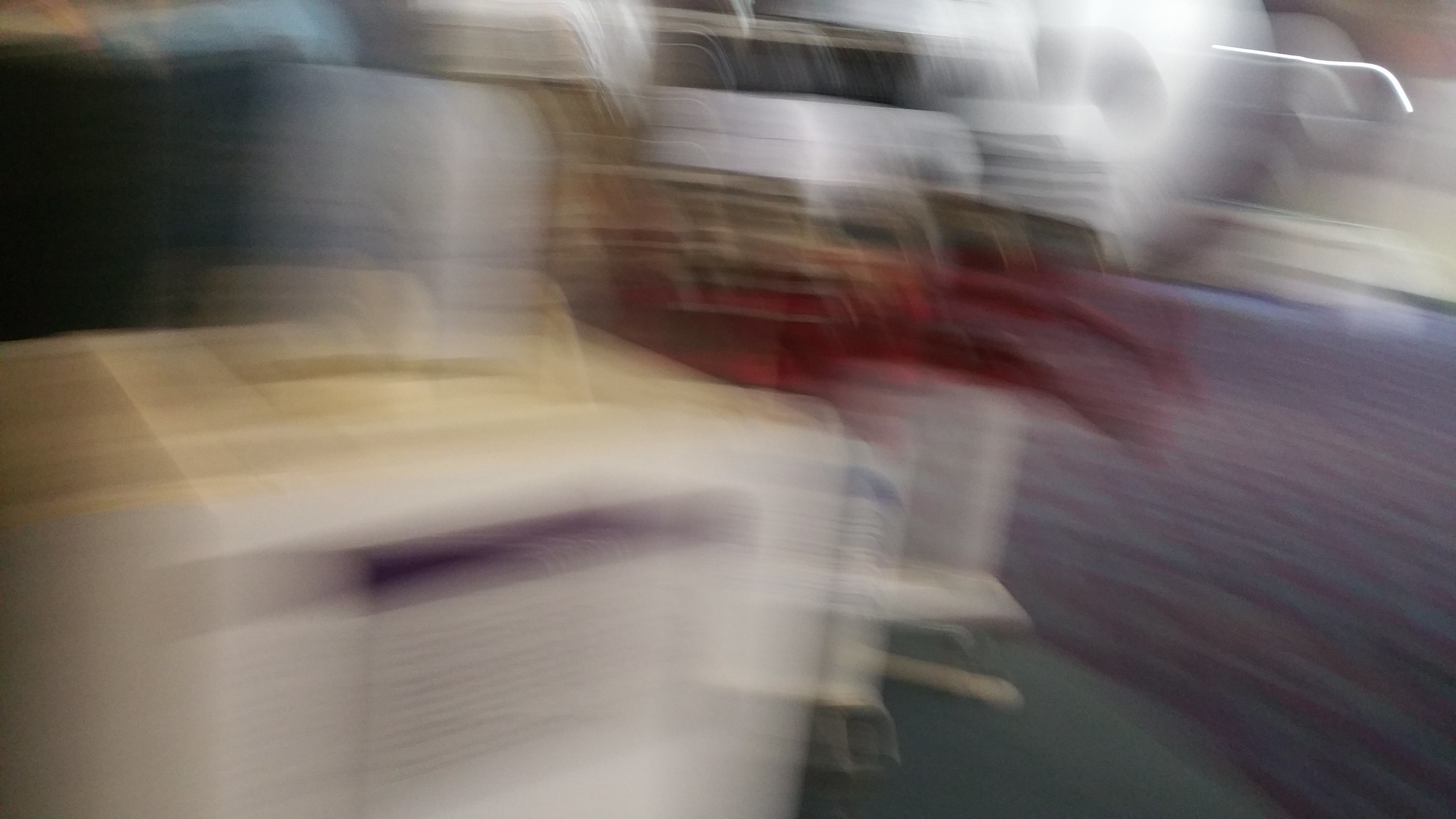In this indoor image, the overall scene is quite blurry with streaks of motion blur running horizontally across the frame. The focal point seems to be a white appliance situated towards the middle left of the image. The flooring consists of a blue carpet with a noticeable red mat laid out on top. More white appliances can be seen scattered in the background. A distinct reflective light can be observed in the top left corner, adding a glimmer to the scene. Various patches of blue, white, and red colors are visible throughout the image, contributing to the overall composition. The space appears to be filled with multiple white reflective surfaces, hinting at a setting with several appliances or reflective objects.